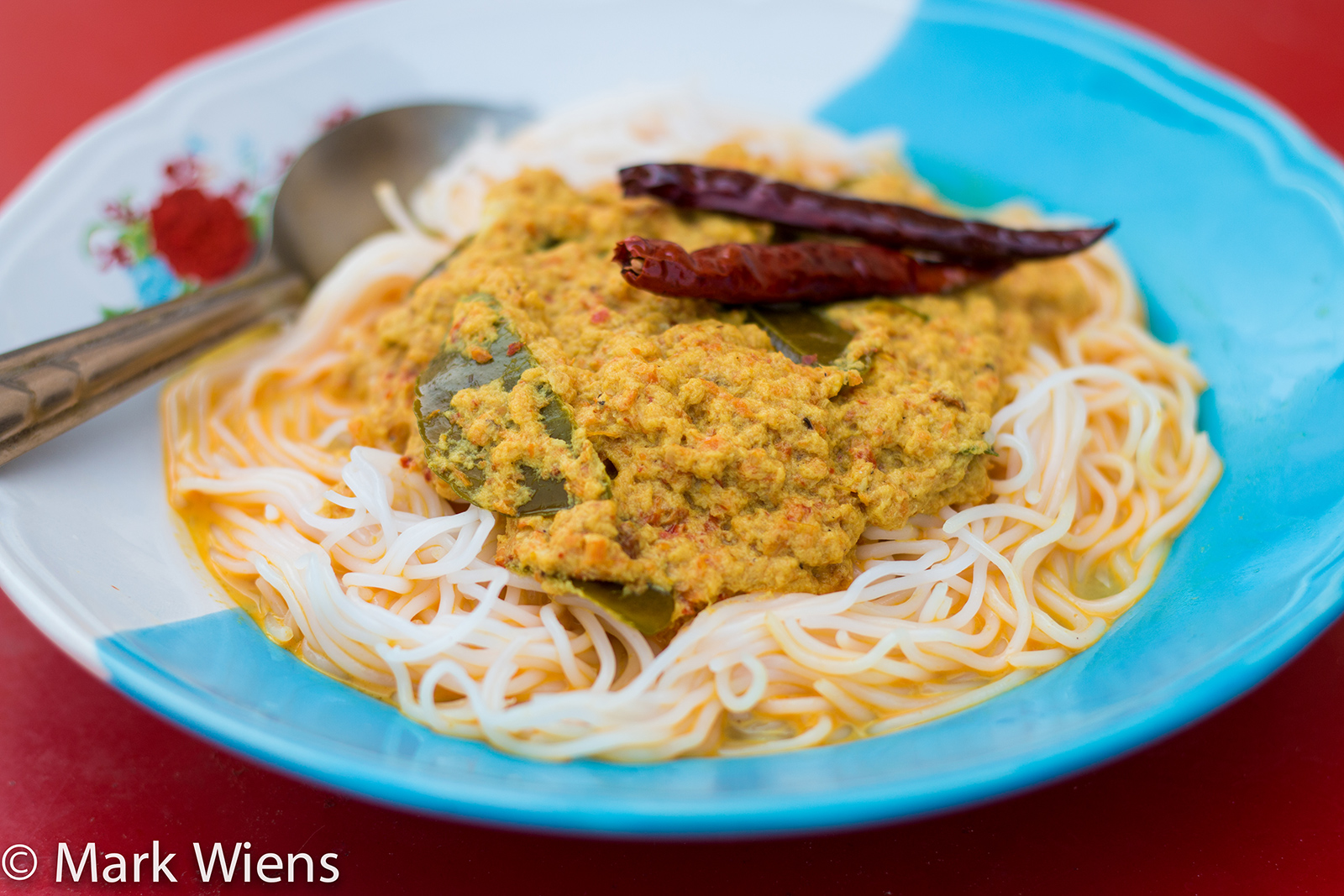This striking photograph, credited to Mark Wiens as indicated by the white copyright text in the bottom left corner, showcases a close-up view of a vibrant meal set on a red tablecloth background. At the center, a half-blue, half-white plate adorned with a floral design captures the eye. The meal itself features white noodles, possibly rice noodles or somen, bathed in a golden curry sauce flecked with greenish-yellow chunks and green mango peels. Topping the dish are two dried red chili peppers, adding a sharp visual contrast. A silver spoon rests on the plate, positioned at the periphery and adding to the intricate composition. The interplay of colors—the deep red chilis, creamy white noodles, and jewel-toned plate against the red background—creates a visually appealing and detailed culinary presentation.